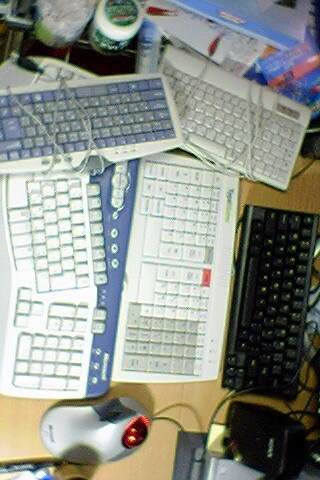In the top-down view of the image, which is roughly one-and-a-half to two times taller than it is wide, a light wooden desk is cluttered with various keyboards. Centered vertically on the desk are three keyboards: at the bottom is an ergonomic keyboard, above it is a predominantly white keyboard with blue accents, and at the top is a gray and white mechanical keyboard with prominent 3D keys, followed by an entirely black mini-styled keyboard.

Above these, arranged horizontally, there are two more keyboards – one of normal size featuring blue, gray, and white colors, and to the right, a smaller compressed version which is off-white. Scattered among these keyboards, there are multiple tangled wires and cords.

In the foreground, there is a silver and gray mouse with a distinctive red button, and to the lower right, another black mouse with numerous connected wires. The background includes a white jar with a green lid, some books, and items covered in plastic. Despite the overwhelming number of keyboards, ranging from black to various shades of white and blue, the image overall has a somewhat disordered appearance.